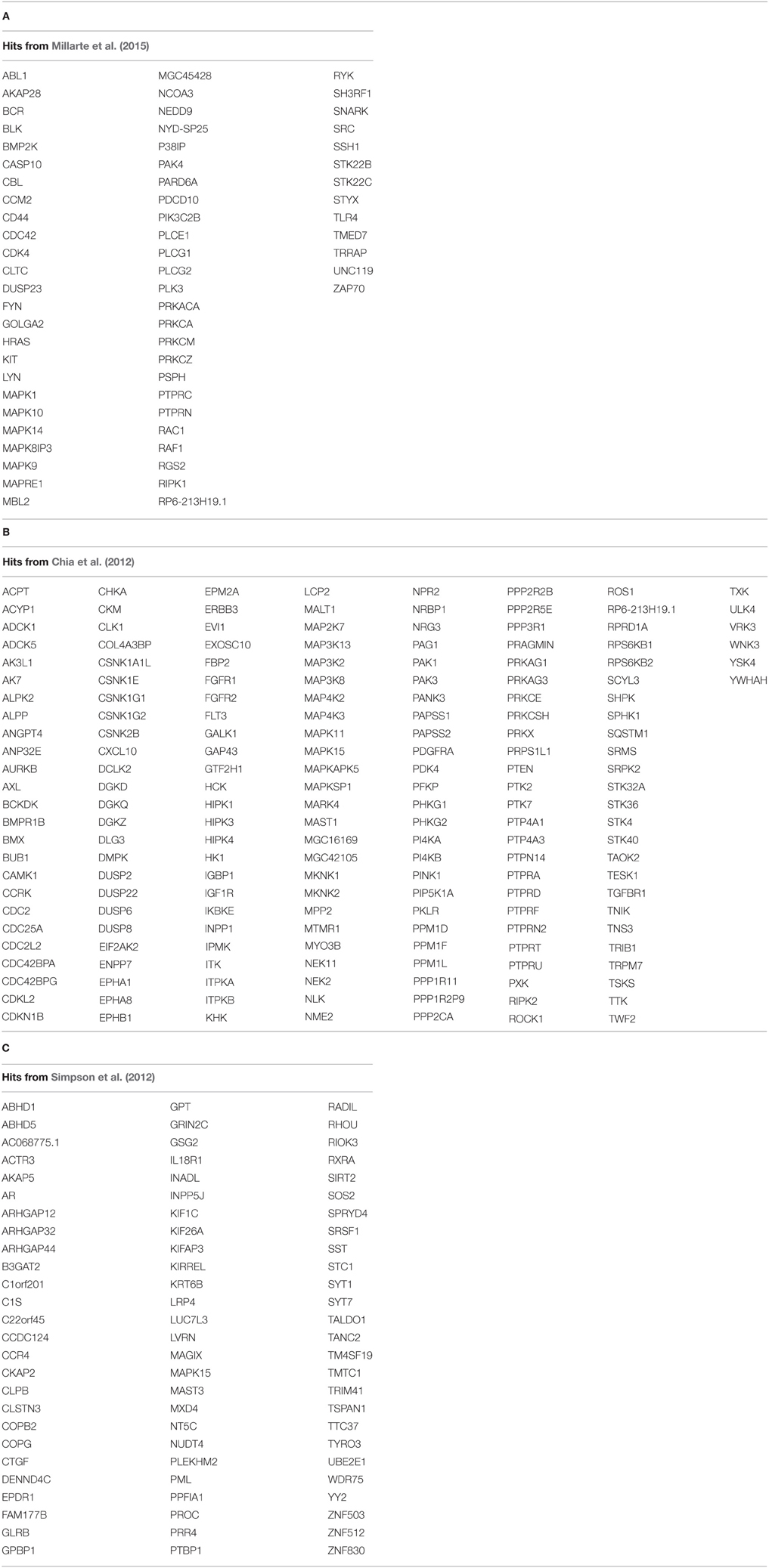This image appears to be a detailed comparative chart from three different research studies, each focusing on a myriad of hits. The chart is segmented into three parts:

1. **Segment A**: This section is based on the work by Millie Arte et al., 2015, with a title "A" above it. It lists a substantial number of hits ranging alphabetically from ABL1 to ZAP70. The text dominating this section is in black color, while the listed items are in a darker slate gray. Light gray lines run across to delineate the entries.

2. **Segment B**: This portion references Chaya et al., 2012, and is titled "B". Here, the hits span from ACPT to YWHAH, suggesting an even broader spectrum of hits compared to Segment A. The text formatting remains consistent with that in Section A, maintaining the black font for the titles and a darker gray shade for the itemized hits, again separated by light gray lines.

3. **Segment C**: Citing Simpson et al., 2012, this segment is labeled "C". Entries in this part range from ABHD1 to ZNF830, presenting a vast array of hits. The styling of the text remains uniform with the previous segments, featuring black titles and dark gray item lists, divided by light gray lines.

The image predominantly consists of a white background with clear, structured text, designed for an informational and comparative presentation. The extensive lists and the methodical alignment of items suggest a thorough compilation of data from multiple studies, though the exact context or application of these 'hits' is not explicitly clear from the caption alone. The combination of black, slate gray, and light gray colors aids in visually organizing the dense information.